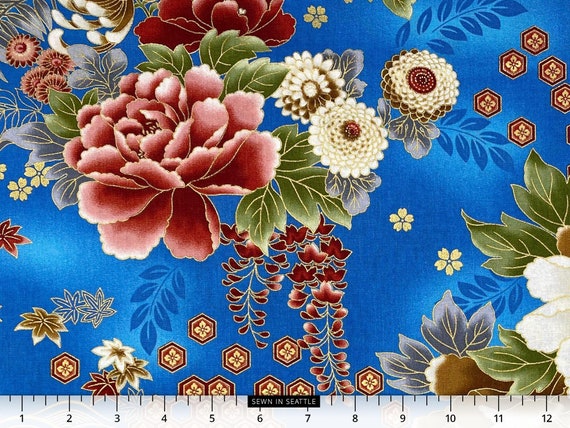The image features an intricately designed brocade fabric with a vibrant electric blue background, showcasing a rich tapestry of floral and geometric patterns. Prominently, there are flowers in shades of wine, silver, white, and gold, adorned with leaves in olive green and silvery gray, all trimmed with gold. The pattern also includes an array of flowers in bright red and delicate white, with notable details such as a large red flower with around 20 petals on the top left and a similarly large, partially visible white flower at the bottom right. Scattered throughout the design are small hexagon shapes resembling a honeycomb, each containing little flowers, adding to the complexity of the pattern. At the bottom, the fabric is labeled "Sewn in Seattle" and features a white, almost transparent ruler measuring 1 to 12 inches, emphasizing the meticulous craftsmanship.